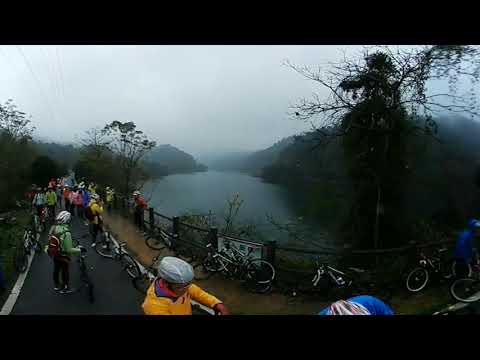This photograph captures a scene of a bike race on a gloomy, overcast day. A large group of cyclists, most wearing helmets and colorful jackets, are gathered on a black paved pathway bordered by grey curbs. The dense crowd is particularly thick on the left side and stretches towards the bottom right corner of the frame. Several cyclists are seen standing with their bicycles, some leaning against a railing or fence, while others have dismounted. In the center of the image, beyond the railing, lies a serene body of water which could be a river or lake, flanked by lush green trees on either side. The background features hills or mountains shrouded in fog, adding to the misty, gray ambiance of the scene. A sign with Asian characters is visible in the middle, with a bicycle parked nearby. The cyclists, including one prominently wearing a bright orange jacket with a white helmet and red gloves, appear to be taking a break, possibly due to the rainy, wet conditions suggested by the cloudy sky and overall damp atmosphere.